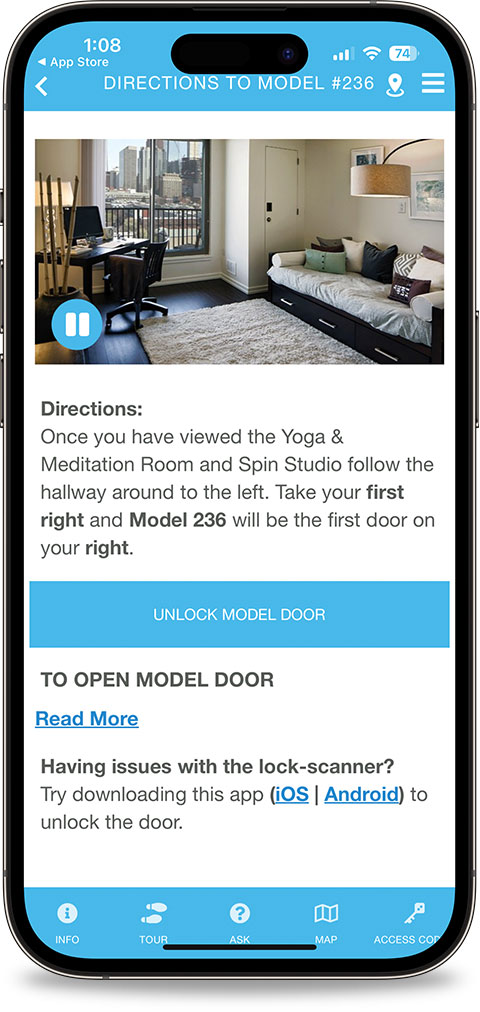The image is a screenshot of a smartphone. The phone’s outline is visible, showcasing a power button on the right side and volume buttons on the left. The device has a blue border at the top. In the top-left corner, the time reads 1:08, with the App Store icon situated below. Moving to the right, four signal bars are visible, with the first three fully shaded in white, along with a Wi-Fi signal and a battery indicator showing 74%.

The central part of the screen displays a heading that reads, "Directions to model number 236" accompanied by a drop pin symbol. Below this, there’s a rectangular picture of an apartment. The apartment view includes a couch against the back wall, a window also on the back wall, and a desk with a computer and a lamp to the left of the window.

Under the picture, instructional text reads, "Directions: Once you have viewed the yoga and meditation room and Spin Studio, follow the hallway around to the left. Take your first right, and model 236 will be the first door on your right." The instructions emphasize the words "right" and "model 236" in black.

Below the directions, a blue rectangular button states, "Unlock Model Door." Further down, a white section labeled "To Open Model Door" contains blue text that says "Read More." This section advises, "Having Issues with the Lock Scanner? Try downloading this app," offering links for iOS and Android to access the app. Finally, it instructs "To Unlock the Door."